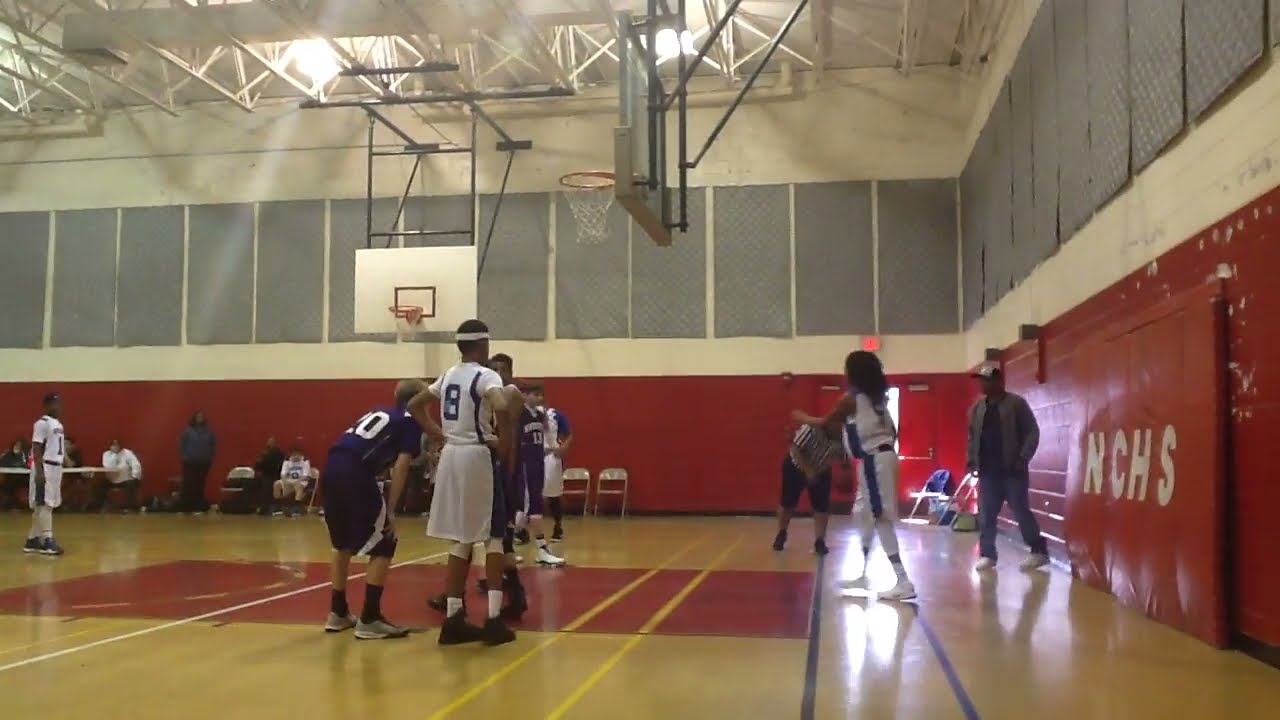The photograph depicts an organized basketball game, likely featuring high school or college-age players, in a large gymnasium or auditorium. The foreground captures the dynamic action of the game, with two teams distinguished by their uniforms: one in white, the other in dark blue. Among the white-uniformed players, a prominent player with number 8 and a headband, who appears to be of dark-skinned ethnicity, faces away from the camera and is at the center of the court. Beside him is another player in white with the number 1 on his back, moving toward the basketball hoop. A third player in white, possibly of Caucasian ethnicity, stands to their left, seemingly observing the action.

On the right side of the image, three players in dark blue uniforms are visible. The player closest to the foreground, with number 21, has dark brown hair and appears to be Caucasian; he is looking off-court rather than focusing on the game. Nearby, a player with number 10 is directed towards the action, while another player further in the background, discernibly Caucasian with light brown hair, also looks away from the center of the court.

The gymnasium's half red walls, accented with a wide white stripe, lead up to tall vertical windows or gray panels, and a ceiling with white metal rafters and bright lighting. The polished wooden floor is marked with classic basketball court lines. Multiple basketball hoops and backboards are visible, including a clear glass backboard with an orange hoop. Near the court’s edge are tables with scoring equipment, an orange-red screen, and seats for spectators and officials, including a referee in a black and white striped shirt. Additional people, likely spectators and staff, are scattered around the court.